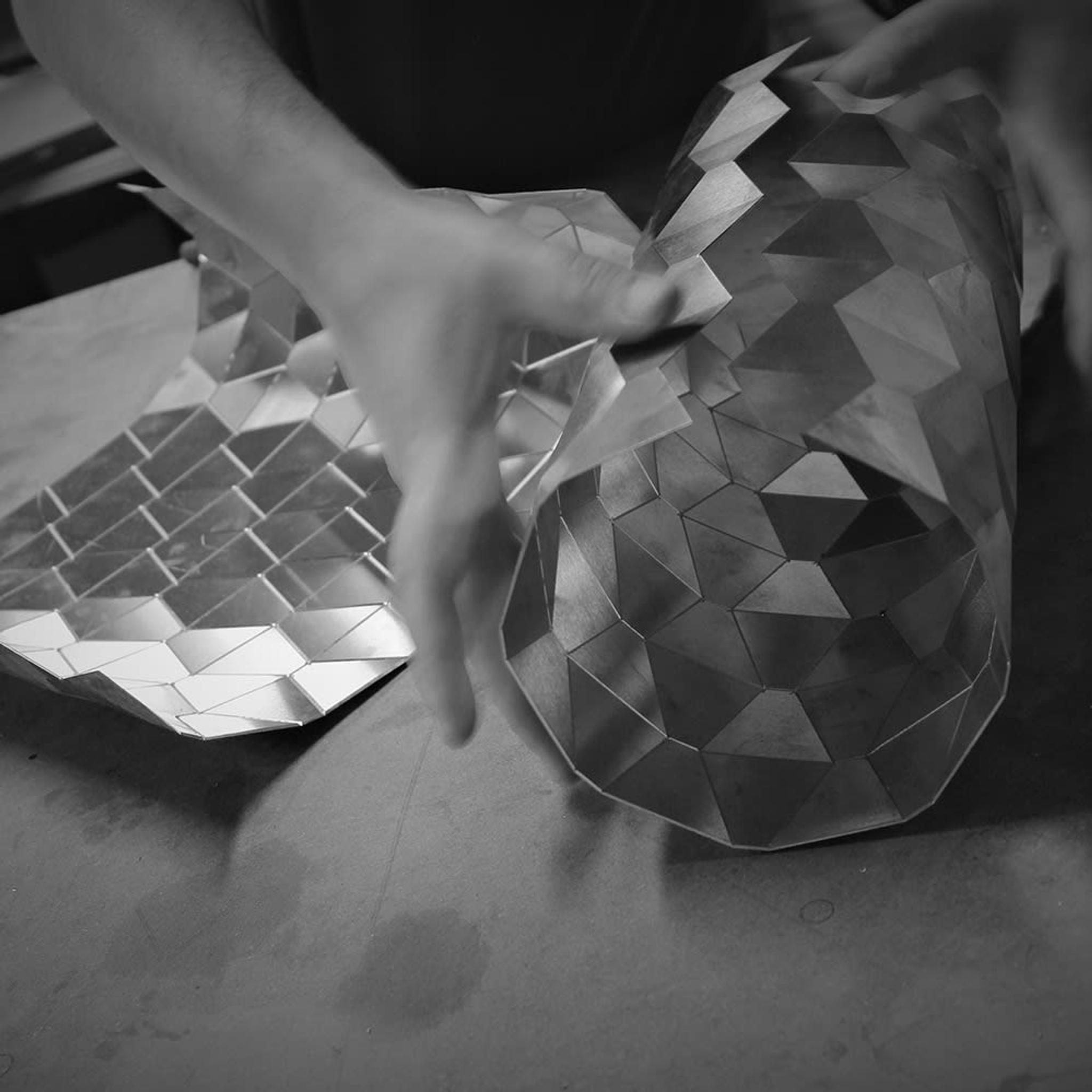In this detailed black and white photograph, a person's hands and a portion of their midsection and right arm come into view, their lighter skin catching the light. The focus is on the individual's hands, which are a blur due to motion, indicating the dynamic nature of the scene likely captured with long exposure in a dark environment. They are meticulously manipulating a cylinder-shaped object made of a reflective, polished material that appears to be either hard plastic or aluminum. This cylinder, adorned with geometric patterns of trapezoids or triangular designs, is being shaped into its cylindrical form. To the left of the cylinder rests another piece of the same material, flat and geometric, poised to be similarly worked on. The entire setup lies on a smooth, flat surface, underscoring the meticulous and artistic nature of this project, suggesting the creation of an architectural model or a sophisticated DIY project.